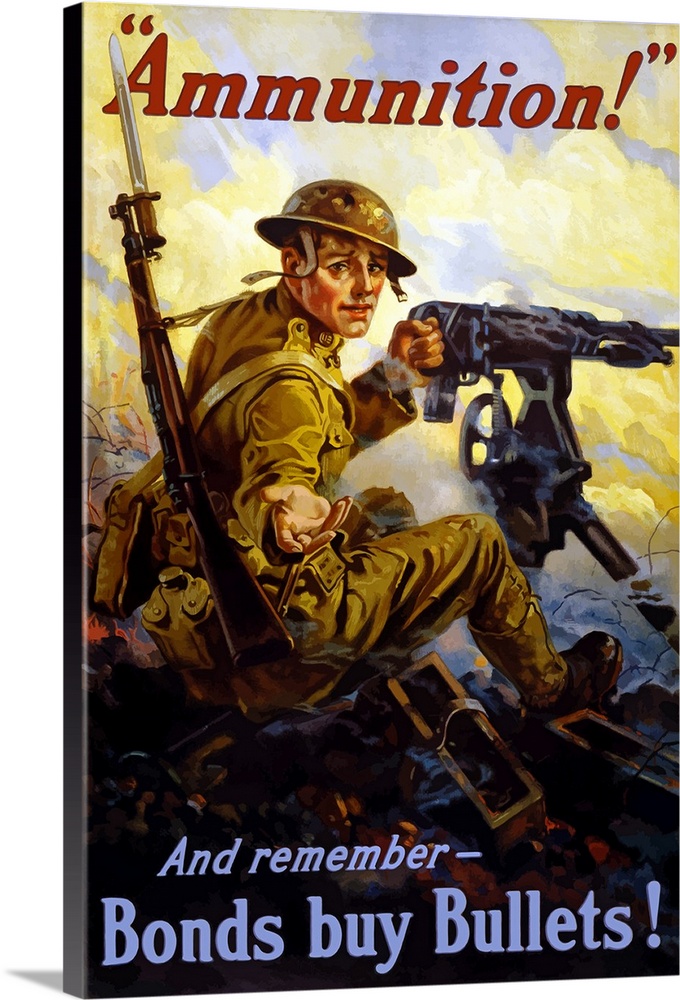This wartime propaganda poster, potentially from World War I or II, features a detailed and evocative illustration aimed at encouraging the purchase of war bonds. The poster, slightly tilted to the right, simulates the appearance of a board or book, casting a shadow behind it for added depth. Across the top, in dark red, capital letters framed by quotation marks and followed by an exclamation point, it reads "AMMUNITION!". This bold title is partially obscured where the bayonet affixed to the central figure's rifle intersects with the first letter.

The central figure is a soldier clad in olive-colored army fatigues, seated on what appears to be a hill, likely within a trench warfare setting. Adorned with a tin hat, possibly indicating World War I era, the soldier grips a machine gun with his right hand while a rifle, complete with bayonet, hangs over his back from a sling. The ground beneath him is brown, further enhancing the gritty, war-torn atmosphere, complemented by a backdrop of a blue sky interspersed with clouds.

Positioned around his feet are boxes suggestive of ammunition. At the bottom of the poster, an imperative message is displayed in pale blue italics: "and remember," followed by non-italicized blue Roman text emphasizing the call to action: "bonds buy bullets!" with an exclamation mark. This compelling composition serves not just as propaganda but as a vivid reminder of the critical role that financial support played in wartime efforts.